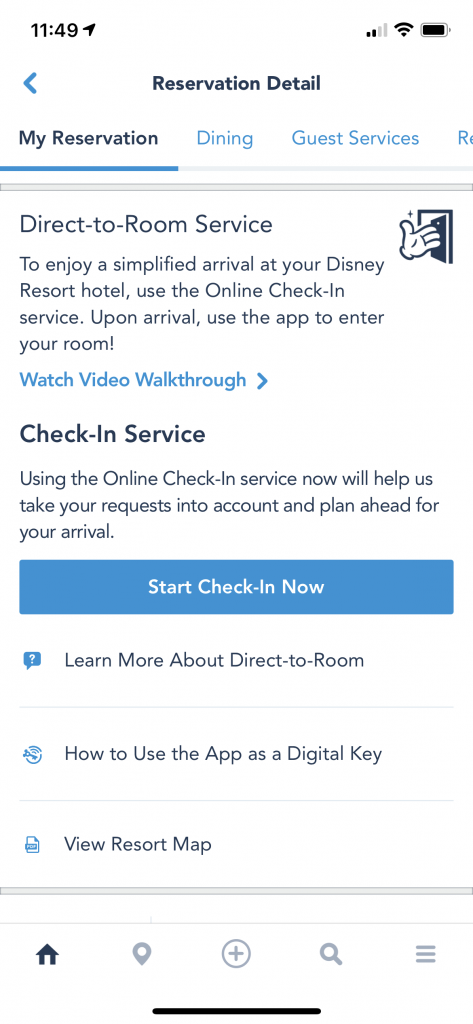Screenshot of the Disney app displaying the "Reservation Detail" section. The section is divided into three tabs: "My Reservation," "Dining," and "Guest Services." The "My Reservation" tab is currently active, with the page titled "Direct to Room Service." A graphic of a Disney glove hand opening a door accompanies the title. Below it, the text describes enjoying a simplified arrival at your Disney Resort Hotel using the online check-in service. Guests are encouraged to use the app to enter their room, with a link provided for a "Watch Video Walkthrough."

The next section is dedicated to the check-in service, featuring a prominent blue "Start Check-in Now" button. Below the button, there are three informational rows: "Learn More," "Direct to Room - How to use the app as a digital key," and "View Resort Map."

At the footer, a navigation bar includes icons for Home, Location, Plus, Search, and Menu (three horizontal bars). The webpage has a white background and header. The status bar at the top shows the time as 11:49 on the left and displays icons for battery, cell phone signal, and Wi-Fi quality on the right.